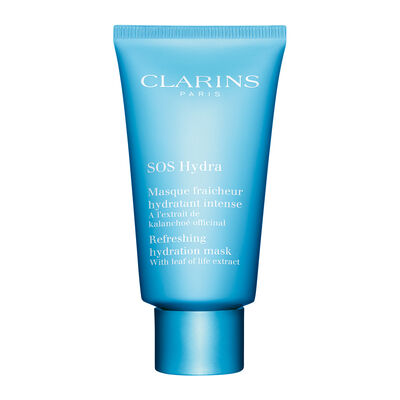The image features a product centered against a white background, creating the illusion that it is floating in a white void. This product is a blue tube with various lines of white text, designed to appear as though it stands upright on its cap, which doubles as a stable base. It's an attractively designed small squeeze bottle, suitable for carrying in a purse. The tube is uniquely shaped: it is wider and more rectangular at the top and tapers to a rounder, narrower bottom. The text on the tube includes: "Clarins Paris," "SOS Hydra," "Mask," "Frasier Hydration Intense," and "Refreshing Hydration Mask with Leaf of Life Extract." The overall presentation is sleek and the minimalist background emphasizes the product, making it ideal for a pharmaceutical shelf or as promotional material.